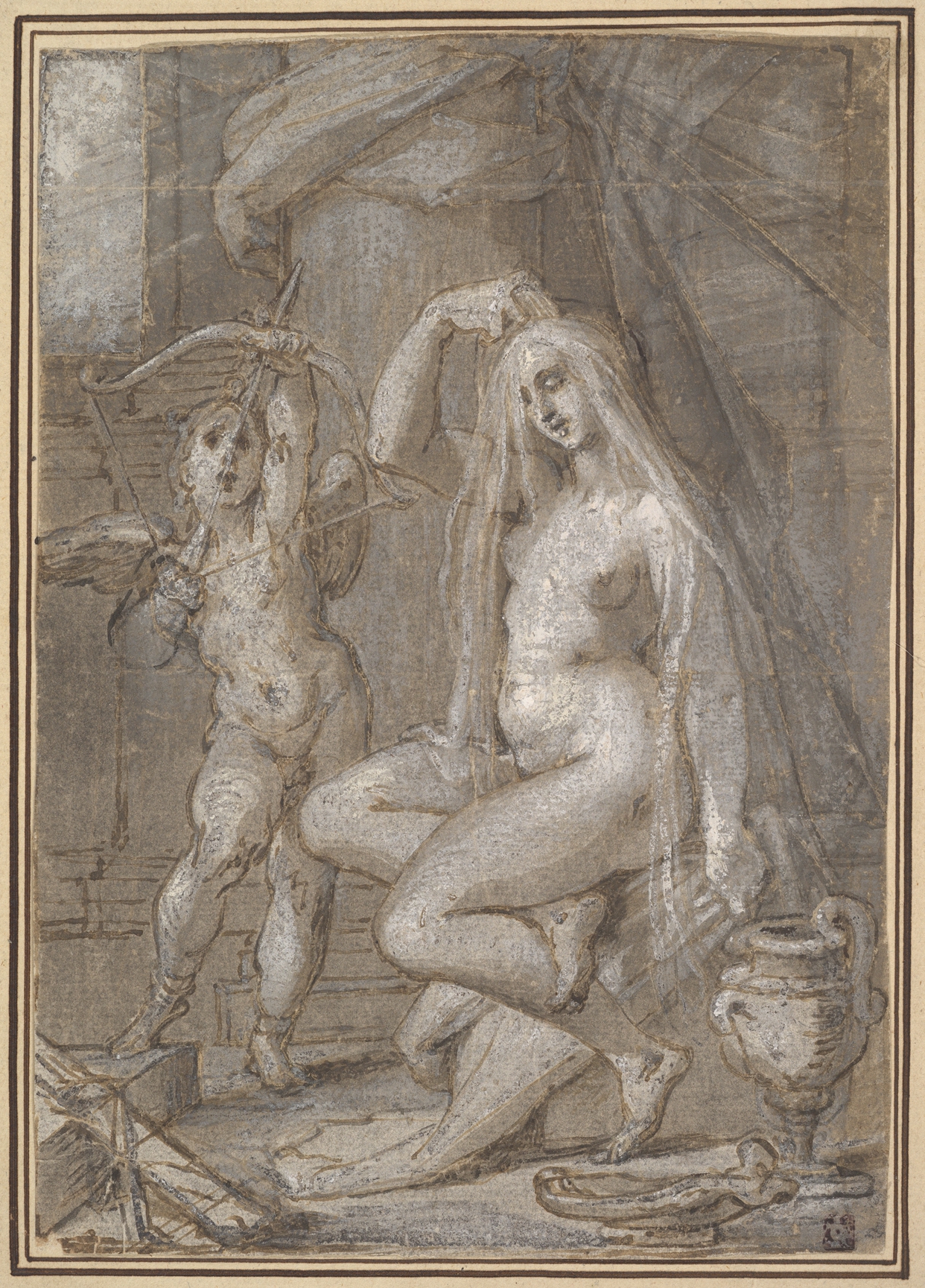This black and white drawing, framed in gold, features a scene with a Cupid and a long-haired woman. The Cupid, positioned on the left, has small wings and is depicted standing with one foot propped on a step. The Cupid is aiming an arrow upward with a bow, using his right arm to pull back the string while looking intently at his target. Directly to the right of Cupid is a nude woman with long hair, parted in the middle and flowing around her shoulders. She is seated cross-legged on a log, her left foot touching the ground while her right foot rests on the back of her left calf. The woman is kneeling and looking downward, with her right arm lifted and her hand touching the top of her head. She wears a long white veil draped over her head. Beside her, there is an urn and a bowl on the floor. A pillar wrapped in cloth stands behind both figures, and a window is visible in the left corner of the scene. The intricate and detailed drawing, although unsigned, emphasizes the interaction between the celestial Cupid and the contemplative woman.